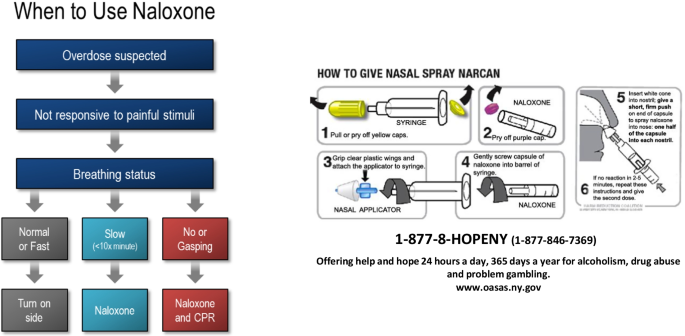This detailed instructional poster on the use of Naloxone, prominently titled "When to Use Naloxone," features a comprehensive decision chart and clear administration guidelines. The left side of the poster, arranged vertically, walks through the steps for determining the need for Naloxone in cases of a suspected overdose. It starts with "overdose suspected," followed by "not responsive to pain stimuli," which directs to assessing the individual's breathing status. This assessment branches into three distinct pathways: 

1. **Normal or fast breathing**: Instructs to turn the person on their side.
2. **Slow breathing (less than 10 breaths per minute)**: Indicates that Naloxone should be administered.
3. **No breathing or gasping**: Directs to administer Naloxone and perform CPR.

On the right side, arranged horizontally, the poster provides detailed, step-by-step instructions for administering Narcan nasal spray. The process includes taking off the yellow and purple caps, gripping the plastic wings, attaching the applicator to the syringe, gently screwing the Naloxone capsule into the barrel, and applying the spray into the nose. These instructions are complemented by illustrative images for clarity.

At the bottom of the poster, a helpline is highlighted: "1-877-8-H-O-P-E-N-Y (1-877-846-7369)," offering support 24/7 for alcoholism, drug abuse, and problem gambling. Further resources are available at www.O-ASAS-NY.gov.